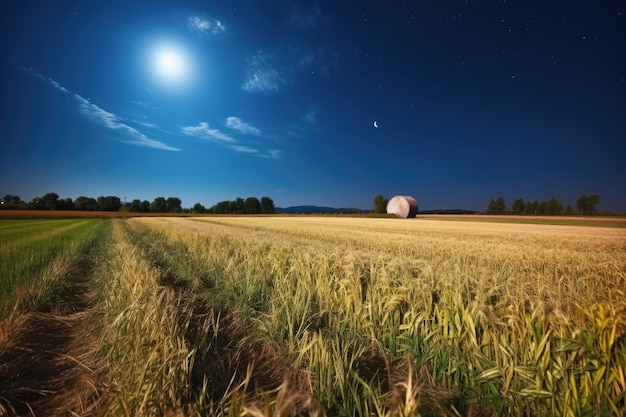In this high-quality photograph of a cornfield taken in the evening, rows of corn stretch symmetrically from the bottom of the image to the horizon, displaying vibrant hues of green and yellow interspersed with brown dirt. At the horizon's edge, a line of puffy, forested trees with large green canopies spans the width of the image. The dark blue evening sky above features several scattered clouds and is illuminated by a luminous, blurred moon, casting a gentle moonlight that almost mimics daylight. On the right side, a cylindrical object, possibly a holding drum, sits at the edge of the cornfield, adding an intriguing element to the serene rural landscape.